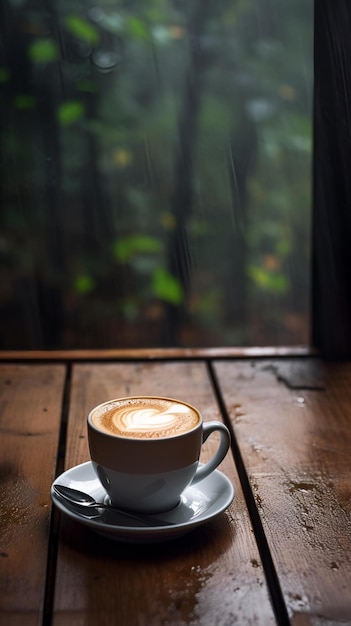On a dark cherry wood surface, possibly an outdoor deck or table, sits an intricate cup of coffee with latte art, featuring a relief design that resembles a leaf or a heart. The white porcelain cup has a distinctive brown top edge and rests on a white saucer. A silver spoon lies in the saucer, bowl up. The surface appears wet, indicating recent rain. In the blurred background, visible through a rain-speckled window, lush green trees and branches add a natural, serene ambiance.